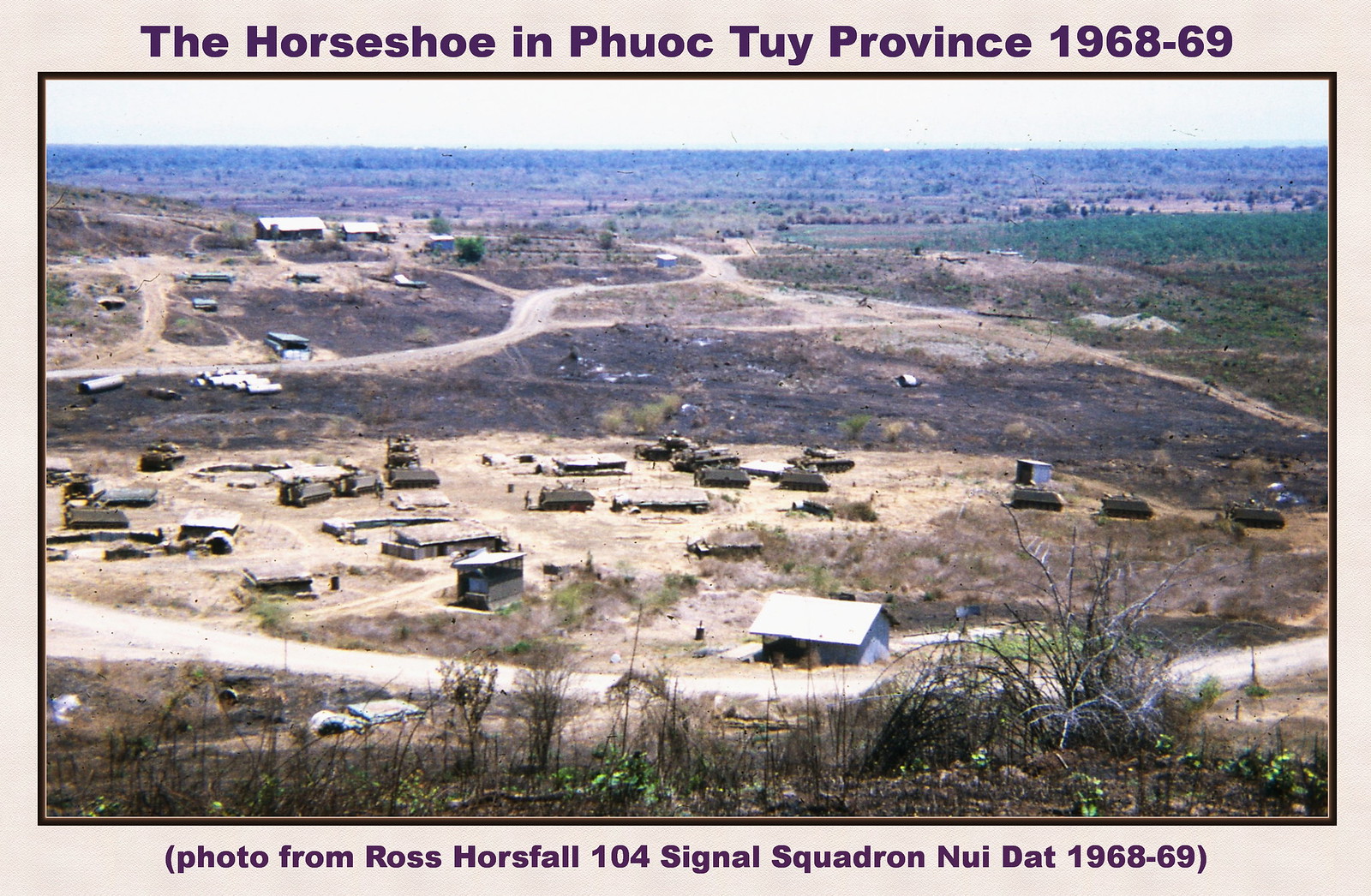The image features a historic photograph bordered by a light tan frame with a darker brown inner border, providing a classic look. At the top of the tan border, dark blue text reads "The Horseshoe in Phuoc Tuy Province, 1968-69." Below the photograph, inside the darker brown border, the text states, "Photo from Ross Horsefall, 104 Signal Squadron, Nui Dat, 1968-69." The photograph itself captures a hillside view overlooking a flat, mostly barren landscape with some green areas and undeveloped sections in the background. Scattered across the dusty terrain are various buildings, large and small, alongside narrow dirt roads. Military vehicles, including APCs and tanks, are parked around these buildings, suggesting an active military presence. The scene appears to be part of a base or outpost, devoid of significant tree coverage, extending towards the horizon.